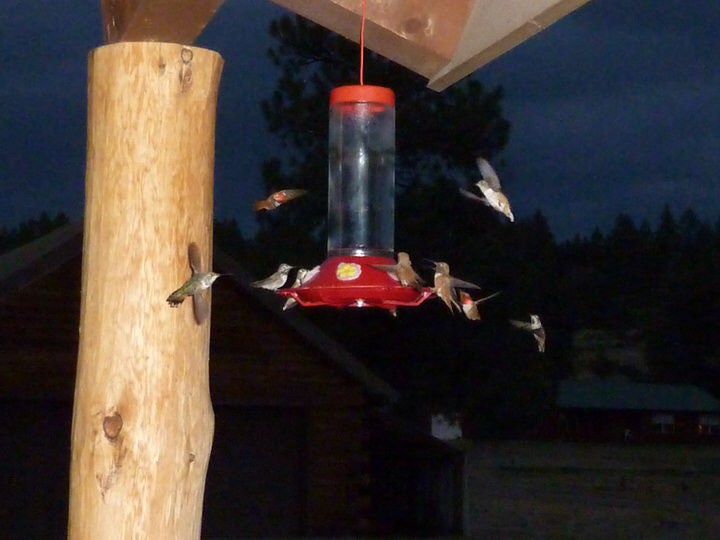In this nighttime color photograph, we see a hummingbird feeder suspended outdoors. The feeder features a clear cylindrical body with a vibrant red top, red strings, and a red base designed for perching. It hangs from what appears to be a wooden structure, possibly a porch, which is partially visible with a hooded roof corner on the left side of the image. Adjacent to the feeder, there is a large, smooth wooden pole standing upright. The background reveals a dark sky and the silhouettes of tall trees and multiple smaller trees, along with shadows of buildings that suggest a residential setting. The scene is bustling with activity as numerous hummingbirds, recognizable by their small size and blurred wings, hover around and cling to the feeder. Their plumage varies, with shades of grey, green, and some sporting red breasts, while one bird appears to be white. The feeder’s translucent plastic makes it difficult to discern any food inside, possibly due to reflections. The hummingbirds are energetically feeding, adding dynamic movement to this captivating nighttime snapshot.